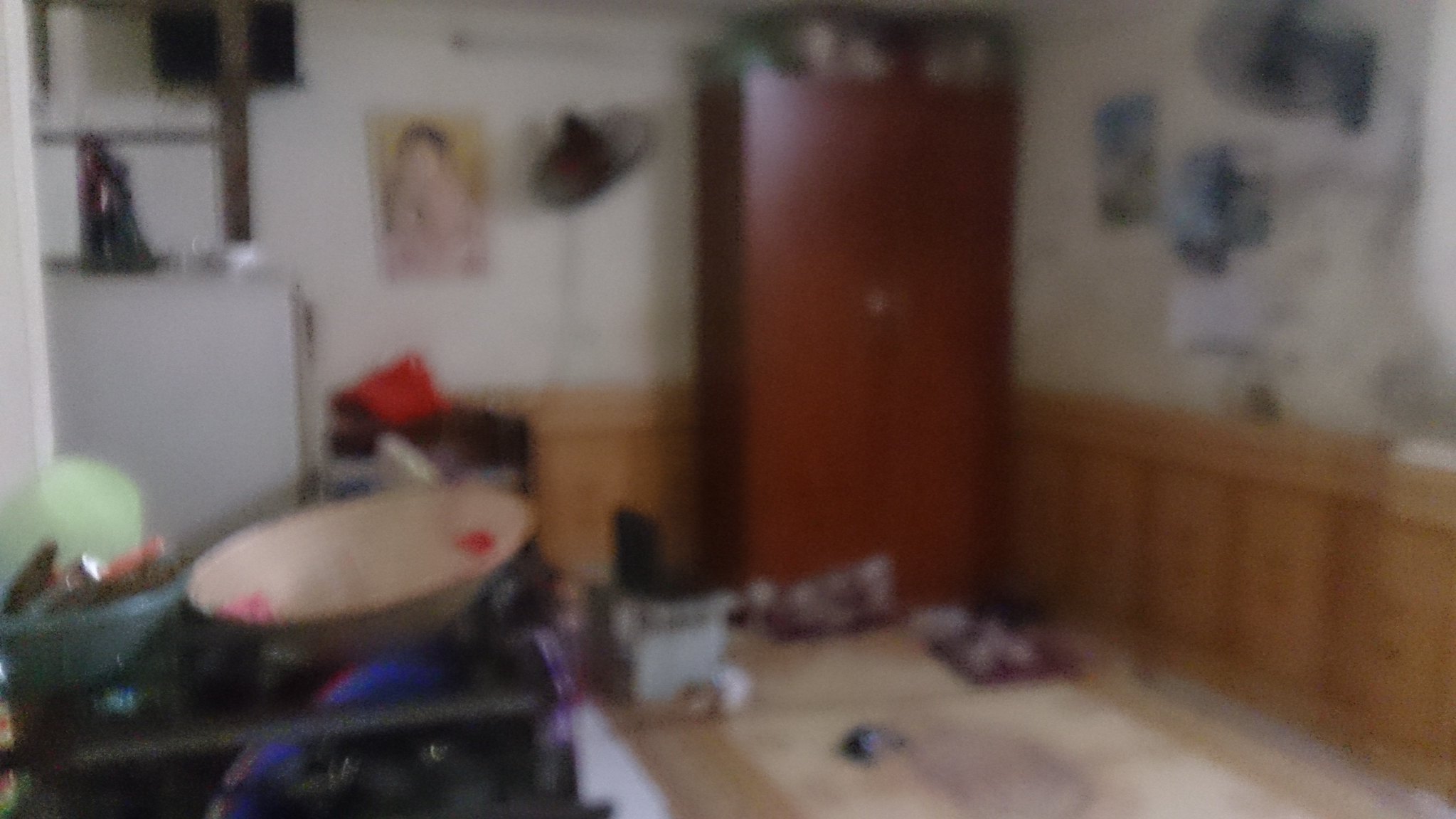The image captures the interior of what seems to be a back room, possibly in a home or a business storage area. Dominating the center background is a large, majestic cabinet crafted from stained wood with a warm, brownish-reddish hue. Atop this cabinet, various items are stored haphazardly. 

The walls are predominantly white, with the lower portion adorned with a wood-like finish. Despite the blur, several calendars are discernible on the walls. The floor is cluttered with indeterminate objects due to the blurriness of the image. 

On one part of the wall hangs a blurred, unframed picture of a child or person, printed on paper. To the side, another cabinet supports a statue, and nearby, a tabletop surface is strewn with an array of bowls, utensils, and other miscellaneous items, contributing to the overall sense of disarray in the room.